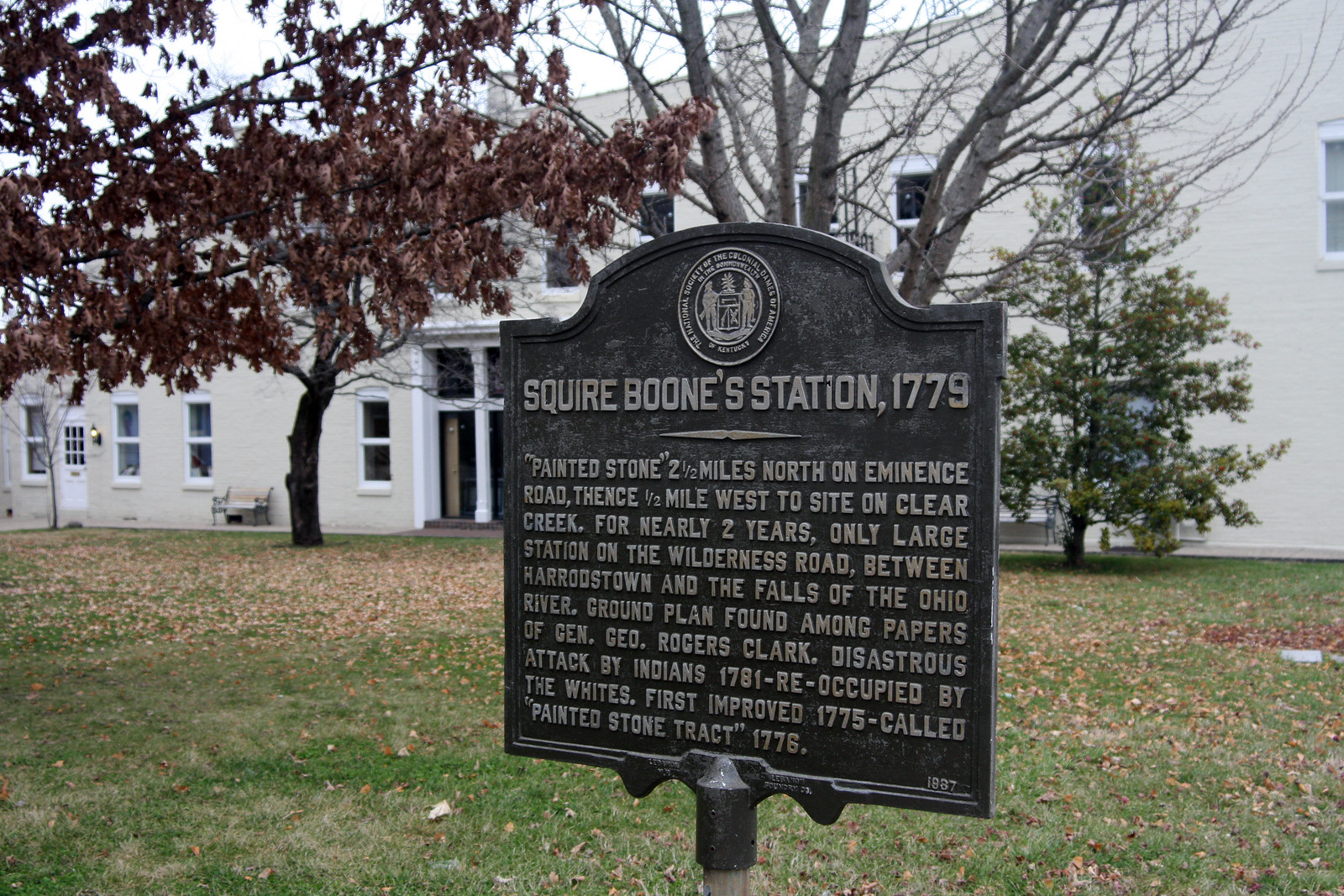In the foreground of this color landscape photograph, there's a detailed historical marker mounted on a metal pole, partially cut off at the bottom, situated in a grassy yard filled with fallen leaves. This marker, presented as a horizontally-oriented rectangle with an arc-shaped top, is made of dark metal with silver-toned lettering. The sign features a circular crest at the top depicting two men and a tree and reads "Squire Boone Station, 1779." It provides historical information: "Painted Stone, two miles north on Eminence Road, then half a mile west to the site on Clear Creek. For nearly two years, the only large station on the Wilderness Road between Heritage Town and the Falls of the Ohio River. Ground plan found among papers of Gen. G.O. Rogers Clark, disastrous attack by Indians in 1781, reoccupied by the whites, first improved in 1775, called Painted Stone Tract, 1778." In the background stands a white two-story building enveloped by trees that are shedding their leaves, contributing to the autumn landscape. A bench is visible on the left of the yard, and the sky above is overcast, adding a muted tone to the scene.